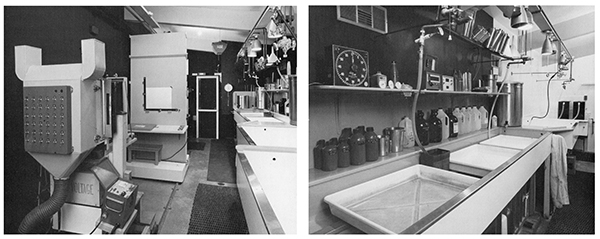The image features a detailed, side-by-side comparison of two black-and-white photographs, both depicting what is unmistakably a professional film photography darkroom. The darkroom is filled with expensive, well-organized equipment, indicative of a highly functional and professional setting. 

On the left side of the image, the darkroom features an enlarging machine, which is a classic tool used in the photo processing workflow involving the use of negatives and light, potentially black light. This section of the room also includes a variety of trays spread across countertops, likely used for different stages of photographic development, and numerous bottles and canisters probably containing the necessary chemicals for processing films.

The right side of the image showcases more of the darkroom’s workspace, including an assortment of heavy equipment and light fixtures casting downward light, suggesting the area is well-lit for precision work. There is a clock with white markings on a shelf, further emphasizing the meticulous and time-sensitive nature of photographic development. White trays, possibly placed in sinks or on countertops, are also visible, reinforcing the assumption that this is a dedicated space for developing photographs.

Overall, the image captures the intricate and organized setting of a film photography darkroom, complete with essential tools and chemicals required for the development process.